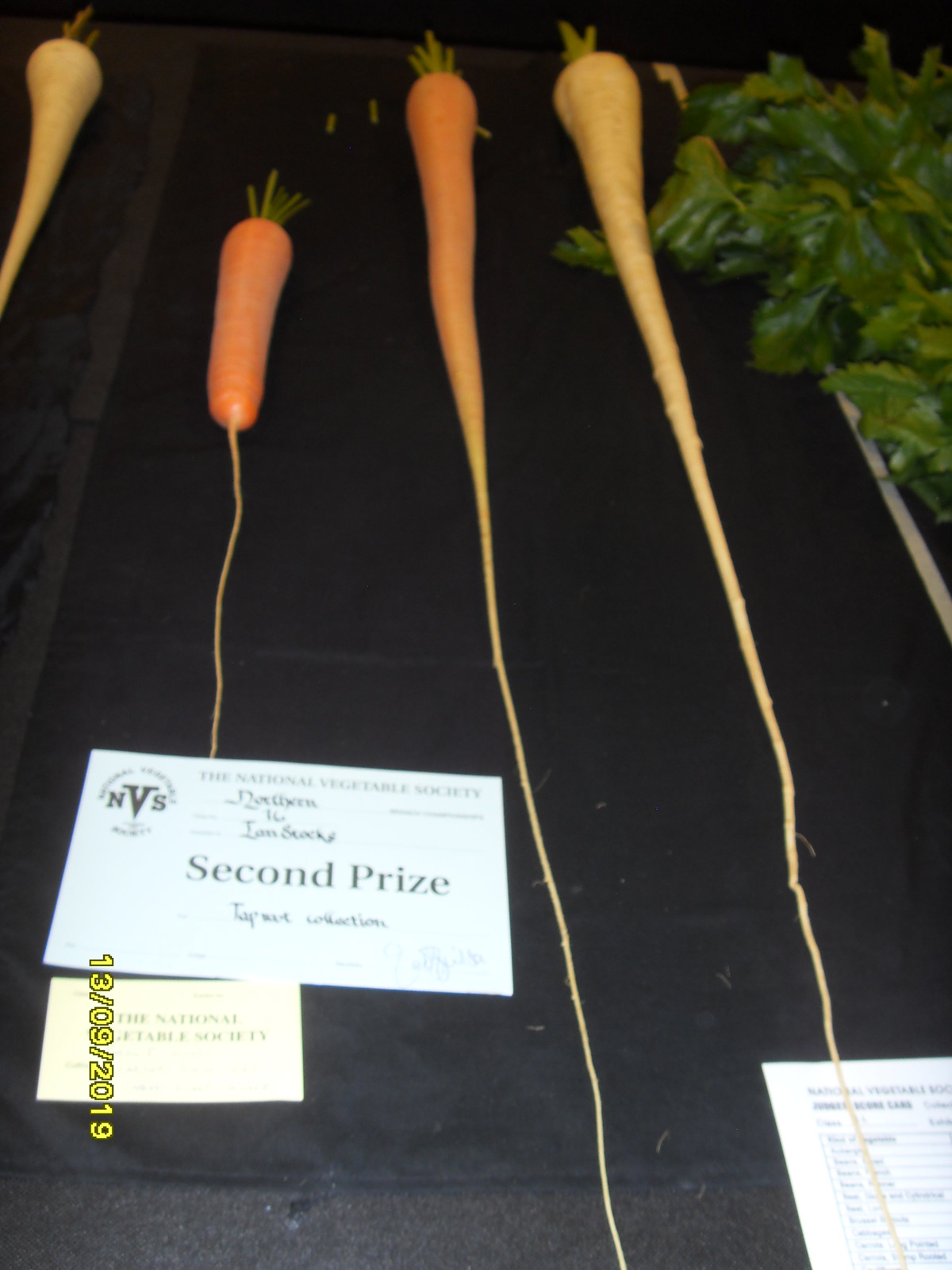The image, taken on September 13th, 2019, depicts a vegetable competition where three orange carrots with notably long roots are displayed side-by-side on a black surface, possibly a table or canvas. The leftmost carrot is unique with its unusually short, plump form and the shortest root, contrasting with the more uniform appearance of the surrounding vegetables. In the bottom left corner, a paper clearly labeled "second prize" from the National Vegetable Society indicates the award status, though other text remains unreadable. Highlighting the setting further are scattered postcards and leafy greens in the upper right, suggesting an arranged presentation for the competition. The photograph has a slight blur, indicative of an older camera, capturing not just the vegetables but a moment of achieved recognition in this 2019 event.